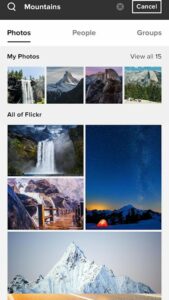This image is a smartphone screenshot of the Flickr website, showcasing its photo-sharing interface. At the top, the black header features the word "Mountains" in white text, indicating the theme of the content. Directly below, a white section presents three navigational options: "Photos" on the left, "People" in the center, and "Groups" on the right, with "Photos" highlighted in a darker font to signify it's the selected tab.

The main content area begins with a heading labeled "My Photos," displaying four stunning landscape photographs. On the far left, there's a captivating image of a waterfall cascading down a mountain. The other three images are equally picturesque, featuring various mountain landscapes; the rightmost photo beautifully integrates trees in the foreground.

Beneath this section, another white border introduces the "All of Flickr" segment. Here, two smaller images on the left showcase different sceneries: the upper photo captures a misty mountain waterfall, while the lower image resembles a painting, depicting a bridge with mountainous backdrops. On the right, a larger photograph dominates the section, characterized by a vast expanse of blue sky. At the bottom of this image, snow-covered mountains bask in the light of either a sunrise or sunset. 

Concluding the page, an expansive image stretches across its width, presenting snow-capped peaks under a gray sky, completing the visual journey through the majestic mountainscapes available on Flickr.